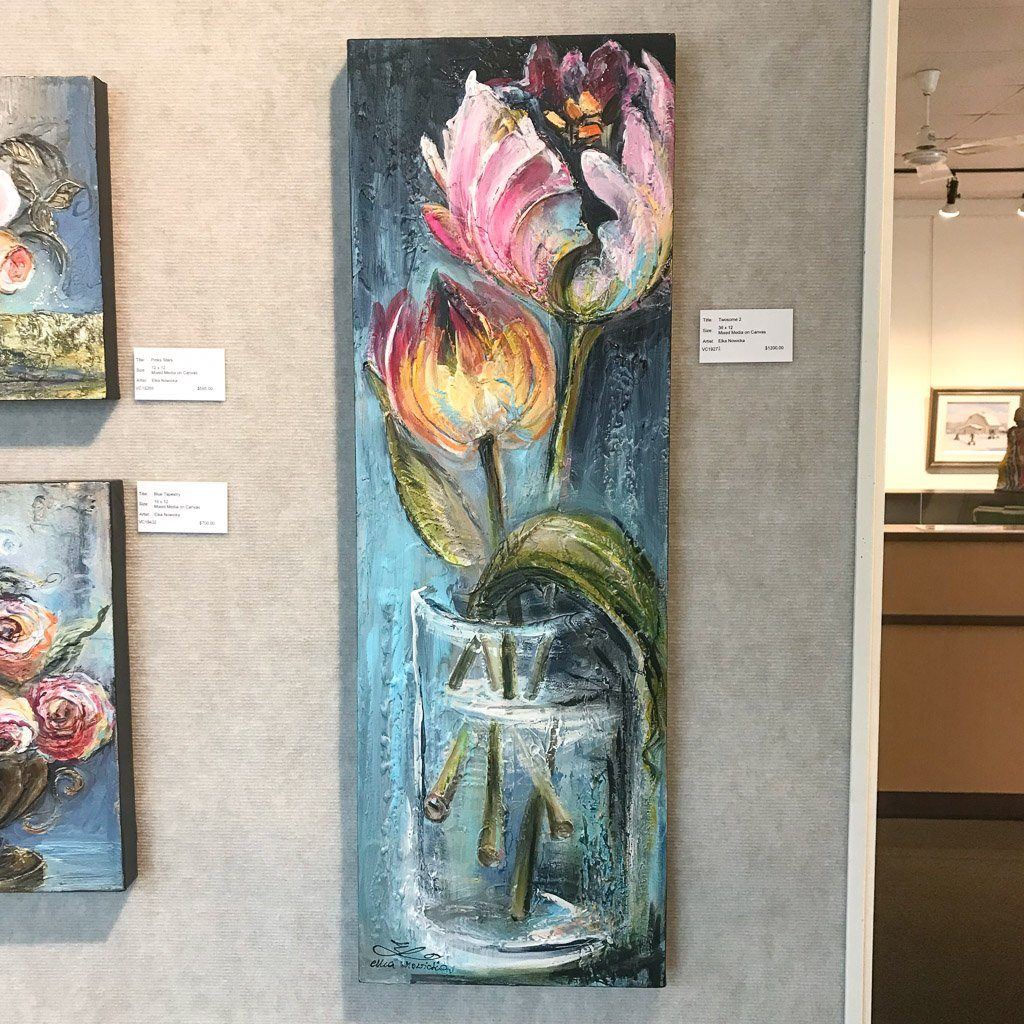The image captures a scene from an art gallery, featuring a gray felt wall with a thin white wood border. Dominating the center is a striking artwork in a vertical triangular frame. This painting, set against a largely blue background, depicts two flowers in a clear glass cup filled with water. The flowers have green stems: one with pink petals and the other with petals that appear orange or golden. On the left side of the main painting are two smaller canvases, positioned one above the other, both showcasing floral designs with varied colors on blue backgrounds. Accompanying each artwork is a white card containing the title, artist's name, and other details. To the right, the gallery extends into what looks like an office or room, featuring a wooden desk, a white wall with an additional picture, a statue on a platform, and a ceiling fan with overhead lighting.